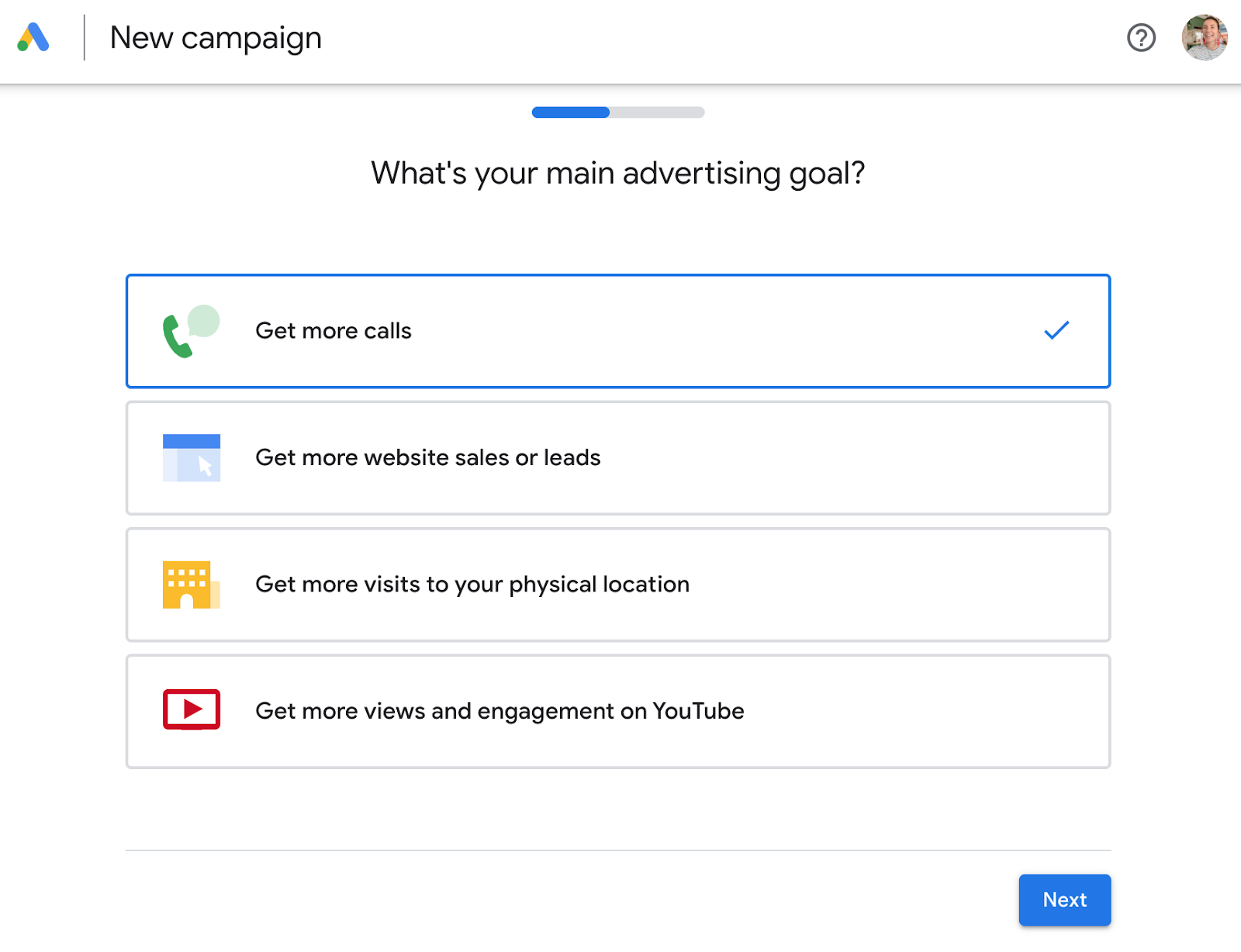The image depicts a screenshot from an online application, likely related to creating a new advertising campaign. The interface has a clean, white background and includes a round avatar located in the upper right-hand corner, suggesting that a user is logged into their Google account. Across the top of the screen, there’s a banner that reads "New Campaign," accompanied by a small logo comprised of a blue, green, and yellow arrow tip pointing upwards. 

Below the banner, a progress bar indicates that the user is nearly halfway through the process, filled in slightly more than a third with blue. The main content of the page is a question that asks, "What's your main advertising goal?" There are four selectable options, each presented in individual boxes with distinct icons:

1. "Get more calls" - represented by a telephone icon and currently selected, highlighted with a blue border and checkmark.
2. "Get more website sales or leads" - represented by a calendar icon.
3. "Get more visits to your physical location" - represented by a yellow building icon.
4. "Get more views and engagement on YouTube" - represented by a YouTube play button icon.

At the bottom of the screen, there is a blue "Next" button, which the user can click to proceed to the subsequent question.